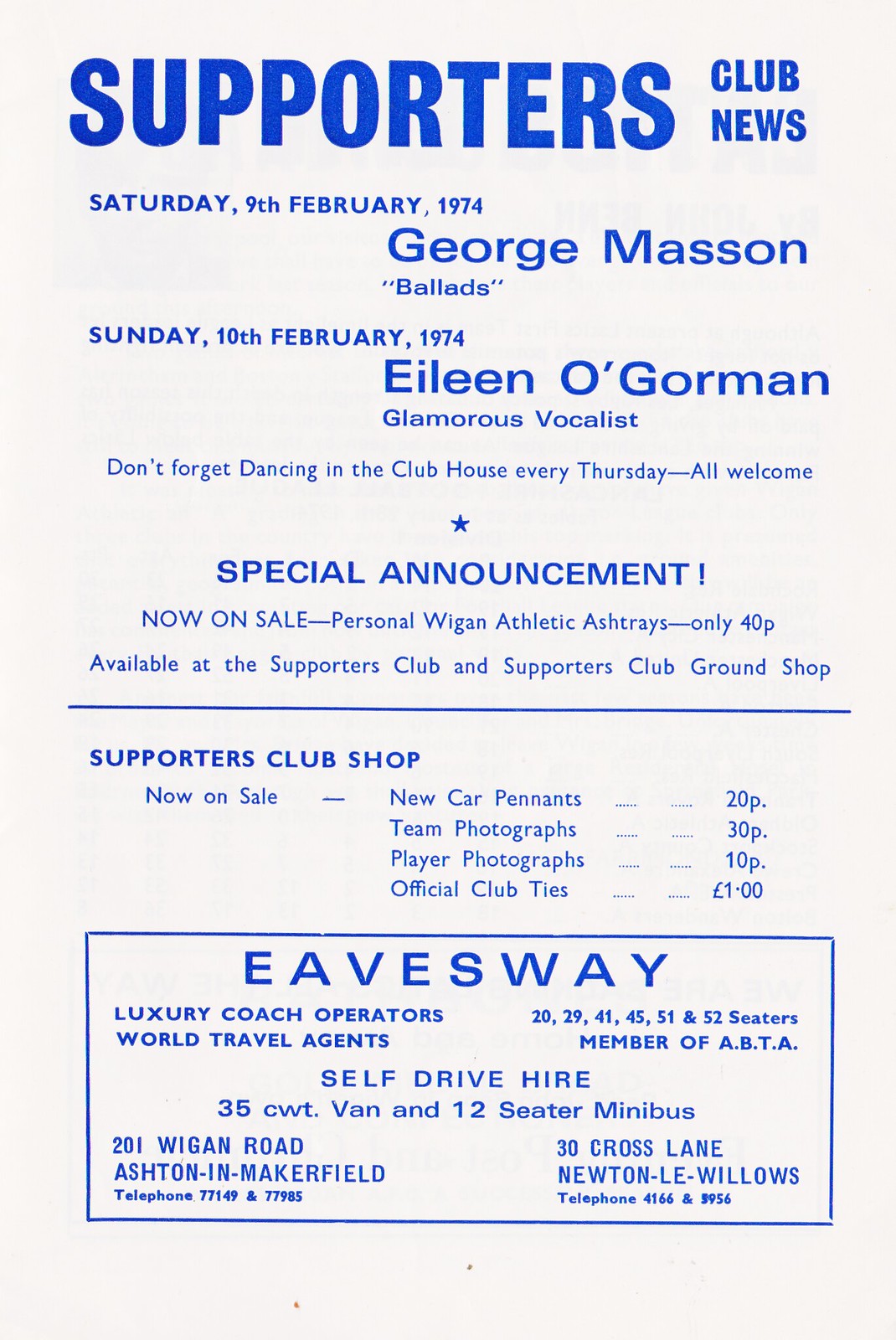This is a photograph of an advertisement or flyer with a predominantly all-white background. At the top left corner, in bold blue letters, it announces "Supporters Club News." Below that, the flyer lists events, starting with "Saturday, 9th February 1974: George Masson (Ballads)." Following this, it details "Sunday, 10th February 1974: Eileen O'Gorman - Glamorous Vocalist." A reminder is then printed: "Don't forget dancing in the clubhouse every Thursday, all welcome."

The flyer features a "Special Announcement" in blue with an exclamation point, stating, "Now on sale: personal Wigan athletic ashtrays, only 40p, available at the Supporters Club and Supporters Club Ground Shop." Below this, the flyer mentions a variety of items for sale at the "Supporters Club Shop," including team photographs. 

At the bottom, within a blue box, it advertises "Eavesway: Luxury Coach Operators" and "World Travel Agents," noting that they are a member of the ABTA and offer self-drive hire services.